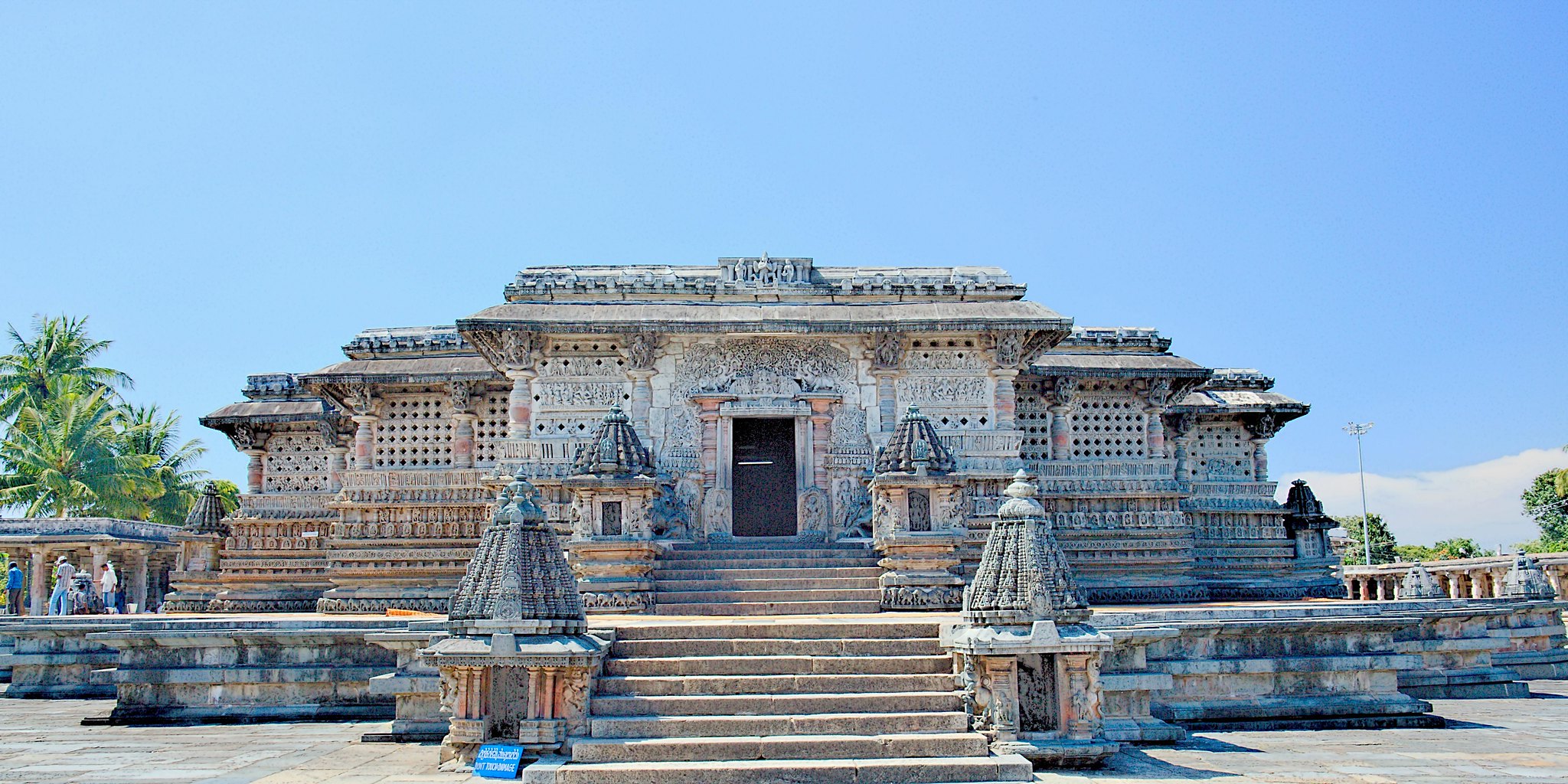The photograph captures an ancient-looking building, likely a popular tourist attraction, as the central focus. The structure appears to be constructed from bricks, cement, and stones, exuding an air of historical grandeur. Leading up to the entrance are two sets of steps: the first set comprises eight cement steps that ascend to a platform, flanked by triangular-shaped pillars—two on each side, positioned at different levels. Another set of approximately eight steps rises from the platform to a darkened doorway, through which the interior of the building is obscured. The facade features small decorative holes that might serve as windows, adding character to the historic edifice. Surrounding the building, the ground is paved with stones. The background reveals a bright blue sky, accented with a few scattered white clouds. To the left of the image, tall palm trees stand gracefully, providing shade to a group of people beneath them.